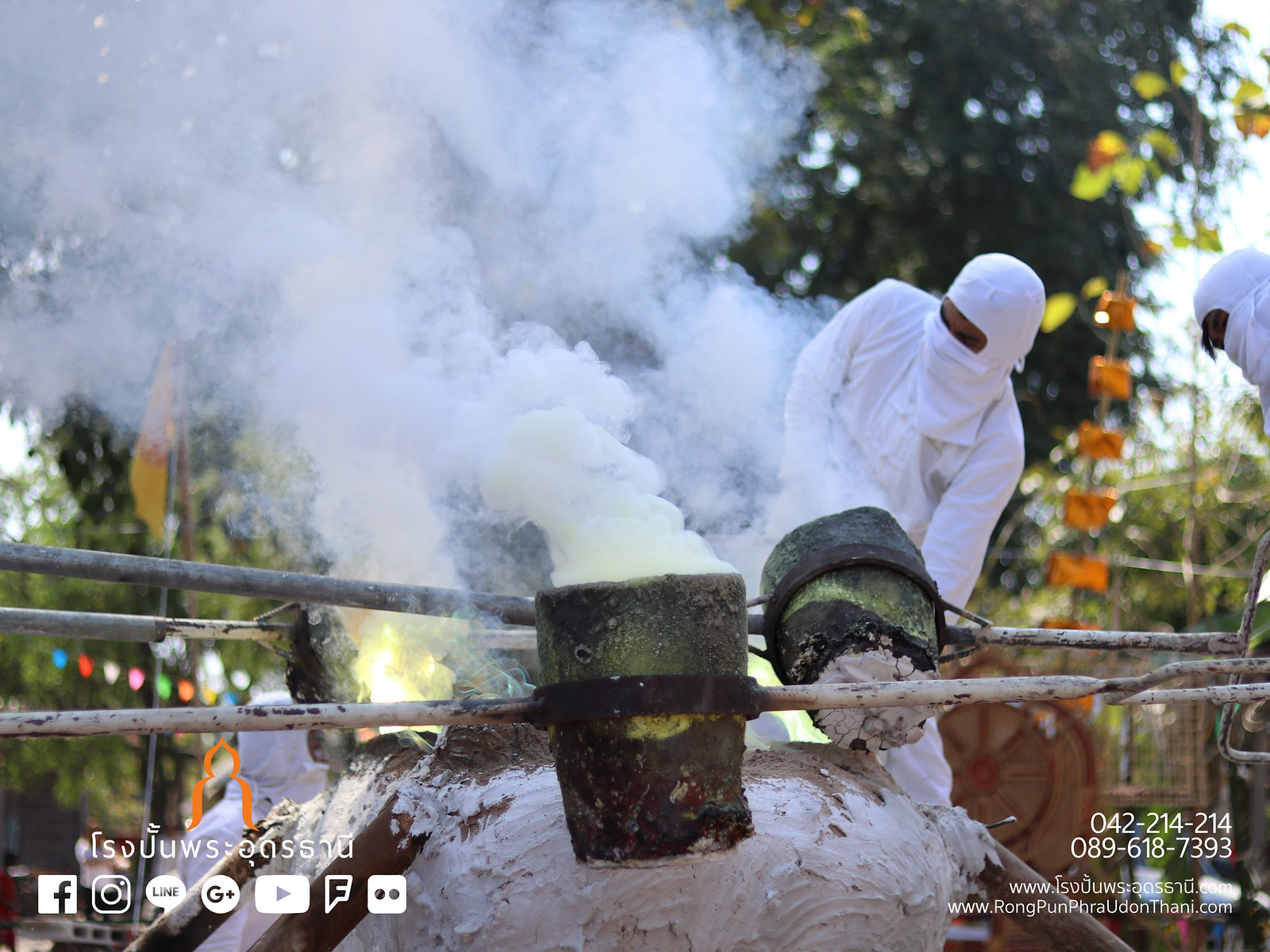The photograph, taken outdoors under a bright sun, captures an intriguing scene centered around a clay fire pit supported by metal bars, with flames flickering on the left and thick smoke billowing upwards. Surrounding the fire pit are two large, rustic green barrels positioned on metal poles. One barrel is being tipped into the pit, emitting additional smoke. At the forefront, white gooey substance is visible, potentially a part of the intricate setup. The scene also features two men dressed entirely in white garments resembling hazmat suits, which cover them from head to toe, leaving only their eyes visible. One man stands prominently behind the fire pit, leaning slightly, while the other’s head peeks from the right edge of the image. Adding to the complexity, three iron bars stretch horizontally across the photo, and the overall background is filled with trees and greenery. The lower corners of the image have various icons and illegible foreign text, hinting at its origin from somewhere in the Far East.